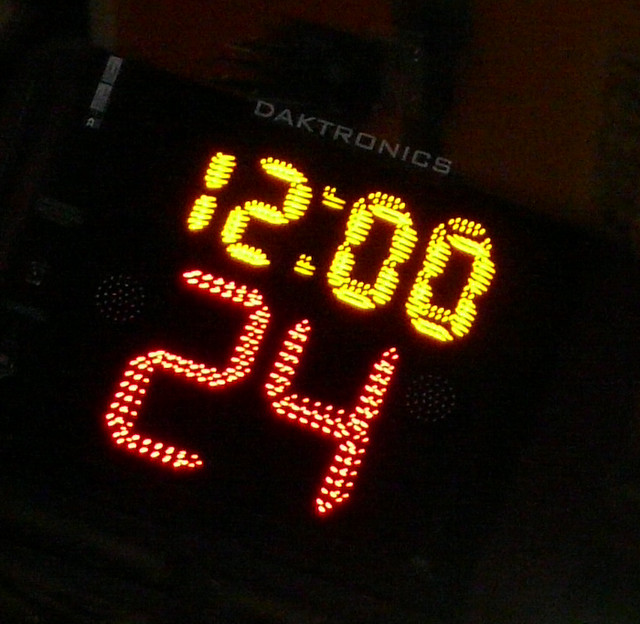The image depicts a close-up, slightly angled shot of an all-black scoreboard. The top of the scoreboard displays the brand name "VACTRONICS" in white lettering. Directly beneath that, a digital clock shows the time as 12:00, with bright yellow digits. Below the clock, the number 24 is prominently illuminated in red. On either side of the scoreboard, there are circular light fixtures that are currently turned off, their shapes faintly visible. The background of the image is very dark and somewhat blurry, with what seems to be a dark brown ceiling or upper wall visible at the top, suggesting the image was taken indoors under low-light conditions.